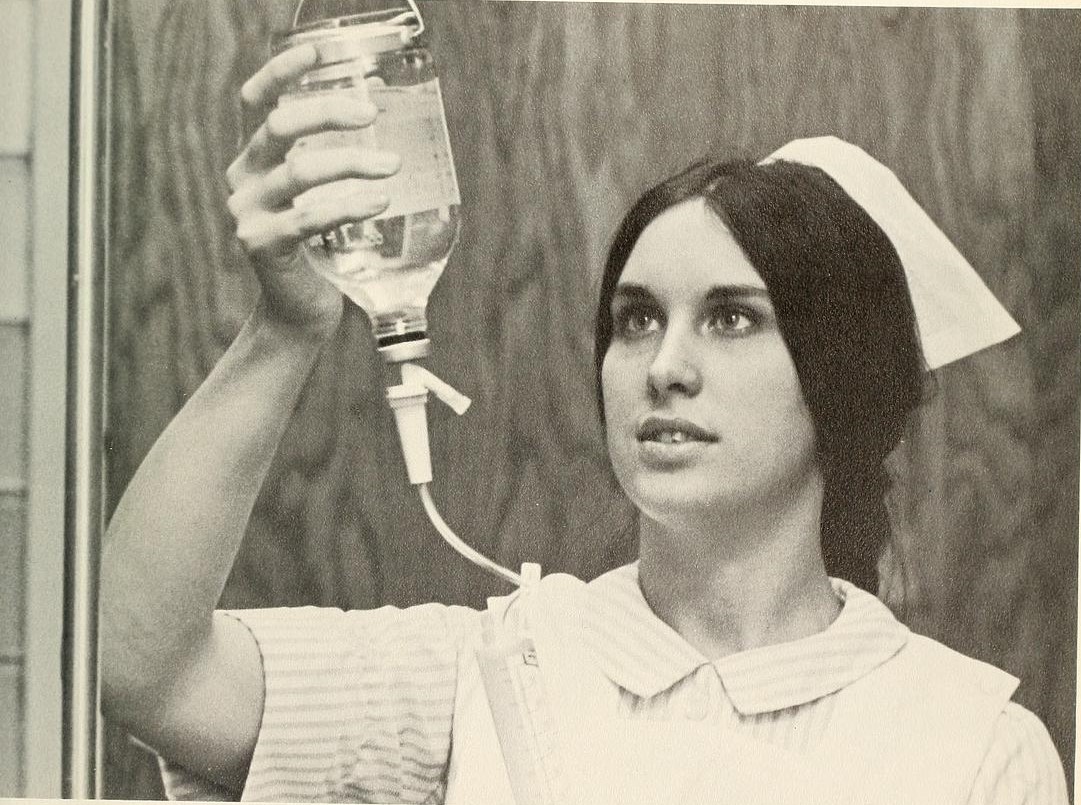In this grainy, black-and-white photograph, a nurse from possibly the 50s, 60s, or early 70s is the focal point. She stands in front of a light-colored, modeled wooden surface, adjacent to a shiny metal rod running vertically through the frame on the left. The nurse, dressed in a traditional uniform, wears a short-sleeved, white-and-gray striped collared shirt along with an old-fashioned nurse's hat that sits atop her long, dark hair, pulled back behind her neck. Her fair skin is notable despite the monochromatic palette. The nurse's gaze is directed upwards and to the left at the object she is holding in her right hand—an upside-down glass IV bottle, with a white cone-shaped piece attached to its end. A white tube runs from this piece down to the bottom of the frame into a translucent syringe or cylinder marked with various gradients. The bottle has a white label facing away from the camera on its far side. She appears to be meticulously double-checking the IV apparatus, all while standing against the backdrop of swirling wood grain, which adds a nostalgic texture to the scene.